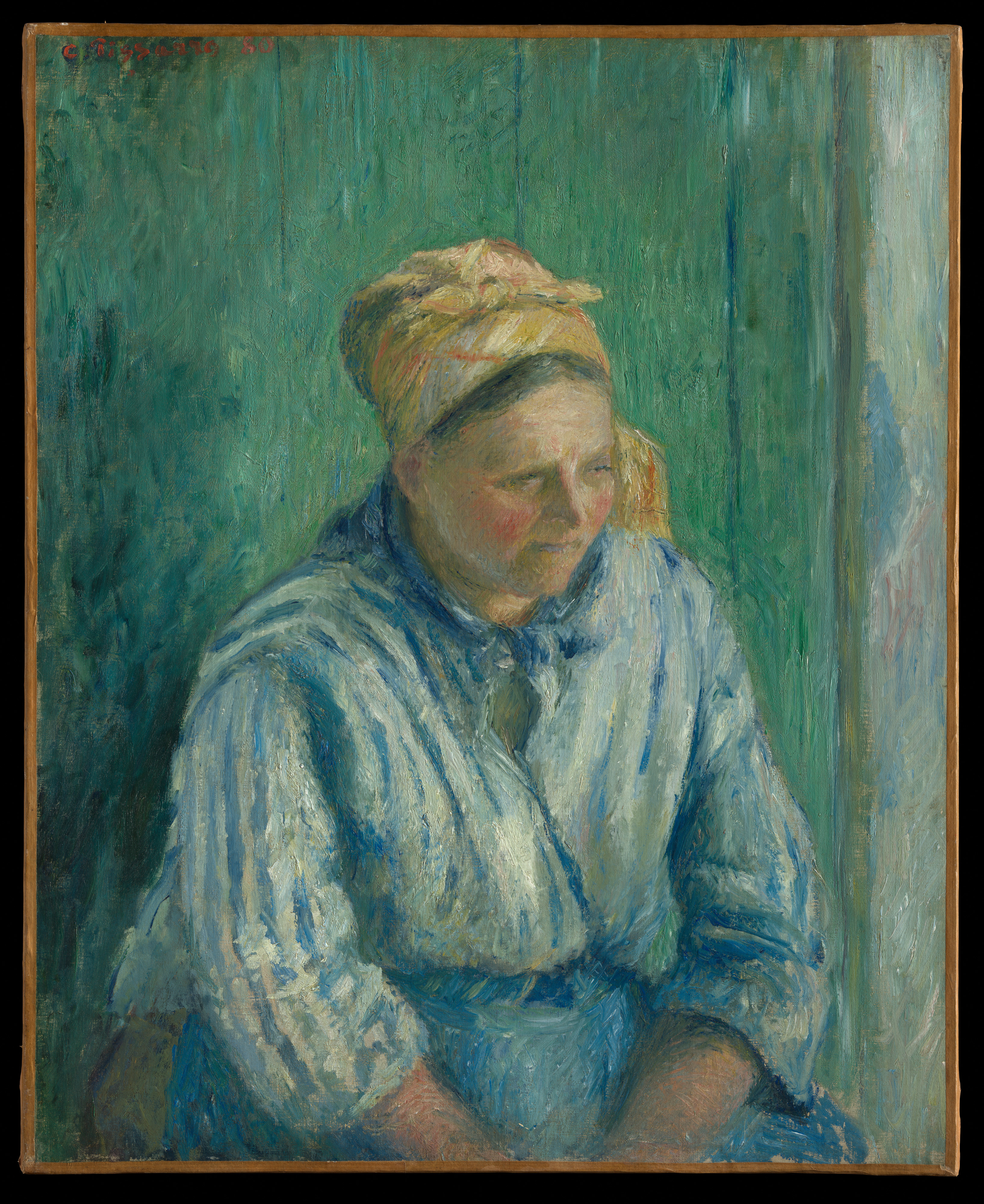The painting depicts a woman seated in front of a closed, vertical green plank wooden door, enveloped in a subtle, grayish-blue haze reminiscent of classical oil paintings. The woman, appearing to be in her 30s or 40s, exudes a sense of fatigue and melancholy. Her dark hair is entirely wrapped in a yellow headscarf interspersed with multicolored patterns, creating a butter-yellow hue around her face. She wears a blue-striped peasant blouse, tucked into what appears to be a brown skirt with a blue apron layered over it. Her rosy cheeks and well-defined nose add to her forlorn expression as she gazes pensively to the right, embodying the ambiance of an old Russian village scene. The entire composition, with its pastel and hazy undertones, bears a resemblance to the works of classical painters like Rembrandt, making it a beautifully crafted yet somber and reflective piece.